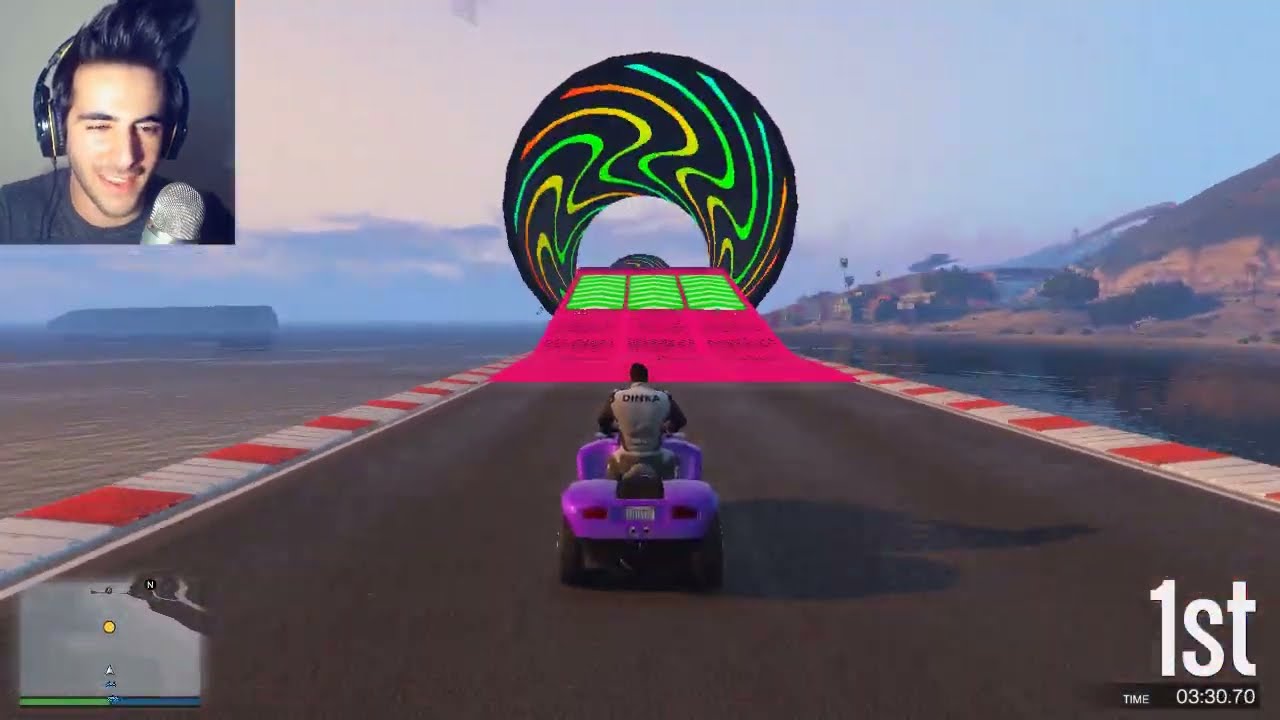The image is a detailed screenshot from a video game. It features a race involving two purple off-road four-wheelers with black tires. One vehicle is launching off a blue metal grid platform suspended in the air, with the other still on the platform. The background highlights a realistic and vividly colored sky, depicting shades of blue, gray clouds, and pink hues, suggesting either dawn or dusk. To the left is a tall mountain range with green shrubs, adding to the scenic backdrop. 

Prominently, in the upper left corner, there is an inset of a person with short, fluffy black hair, wearing a black t-shirt, a headset, and a microphone, indicating they are gaming or live-streaming. Behind this individual is a plain wall. Overlaying the in-game scene, the bottom left corner of the image includes the text "recording" and "MUYSKERM," possibly the player's username, indicating they entered first. The bottom right of the screen shows the text "second" and a timestamp of 4:26:56, implying this could be a timed racing game.